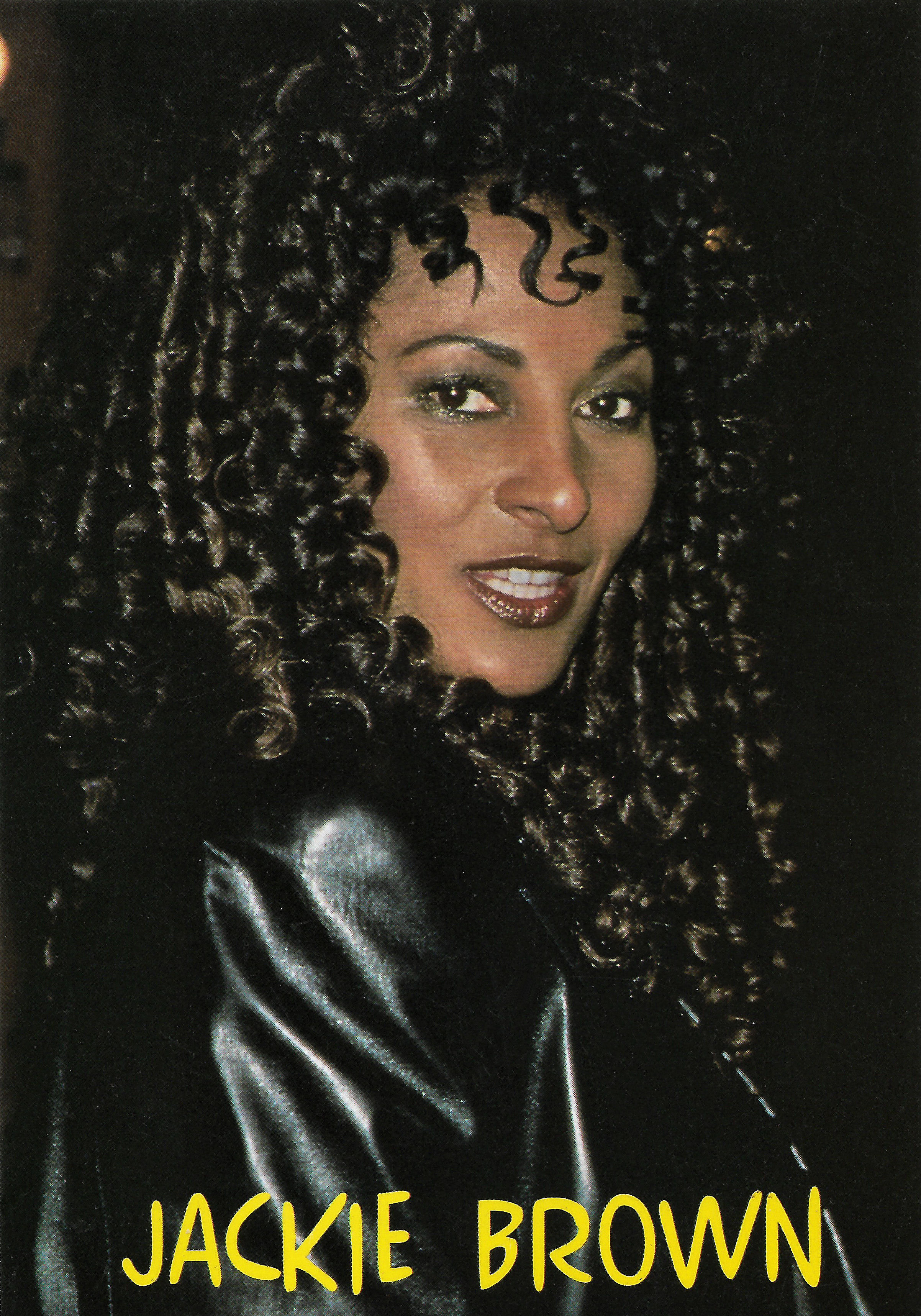The image captures actress Pam Grier, as seen in her iconic role in the 1997 film "Jackie Brown," indicated by the yellow text "Jackie Brown" at the bottom of the picture. Pam Grier is looking directly at the camera, her head slightly turned to the side. She is adorned with shiny dark red lipstick and sparkly brownish-green eyeshadow, enhancing her expressive features. Her long, curly hair cascades around her shoulders, some strands reaching chest level while others fall to shoulder length. She is dressed in a sleek black leather jacket. The photograph has a black backdrop, illuminated by a faint red light in the top left corner and another yellowish glow around her hair on the right, suggesting the image was taken at night, possibly outside near streetlights. Grier’s subtle smile and confident pose convey a captivating presence, making the image both striking and memorable.